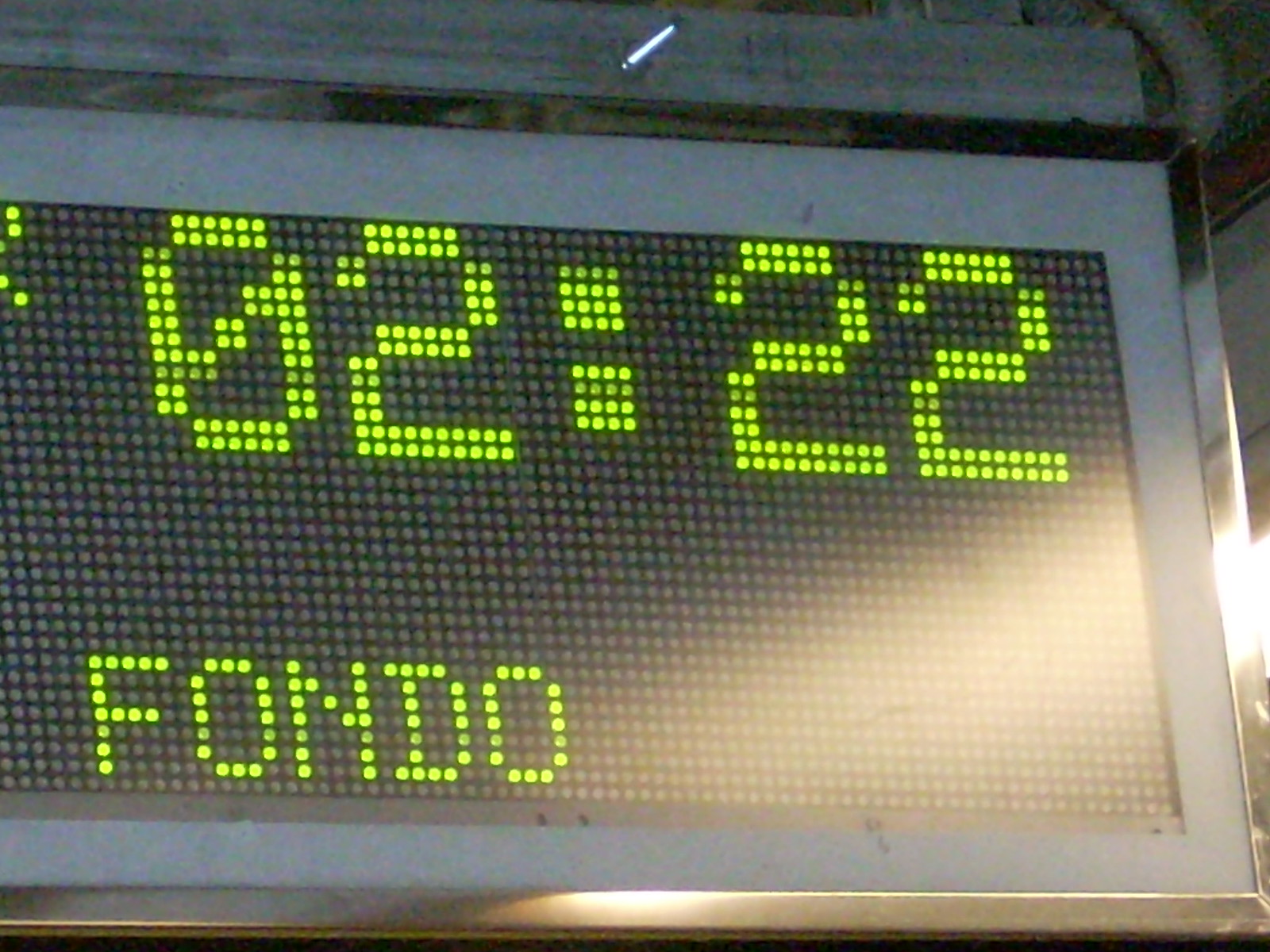A photograph showcases a digital signboard with a sleek gray steel border. The signboard features a black background embedded with small, evenly spaced gray dots capable of illuminating in various LED colors. In this image, the LEDs are glowing a vibrant neon green, displaying the time "02:22" above the word "FONDO" in bold, uppercase letters. The setting appears to be an environment similar to an airport, where clear visibility from a distance is essential. Overhead, gray rafters and exposed gray ductwork add to the industrial aesthetic of the scene.